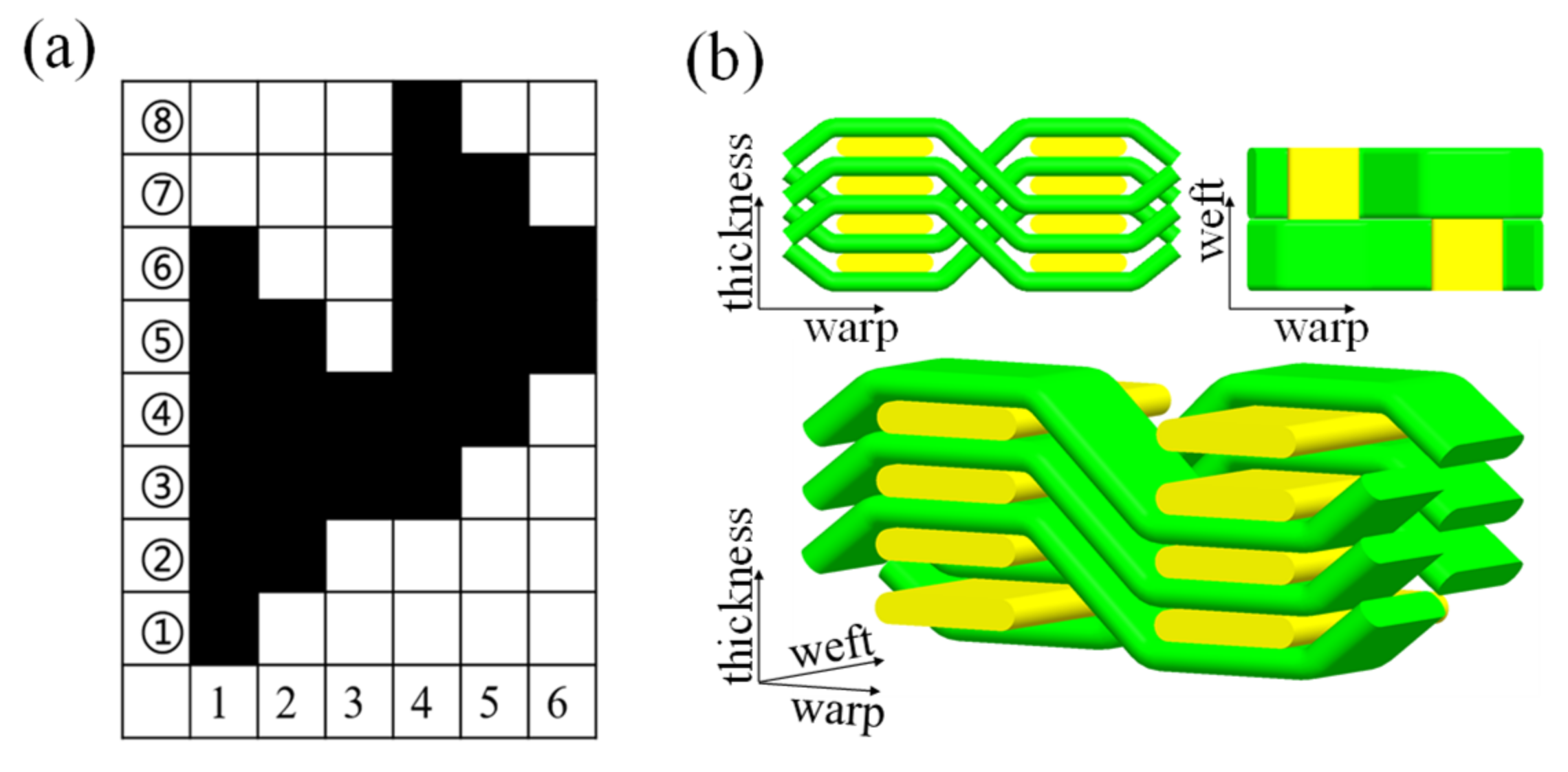The composite image displays diagrams labeled A and B, each serving distinct purposes in illustrating a weaving pattern and its resultant characteristics. 

**Image A** features a 6x8 grid, reminiscent of a crossword puzzle, where rows and columns are delineated by numbers. The grid contains both white and black squares, suggesting a pattern typically associated with weaving diagrams. On the left side of the grid, numbers 1 through 8 are arranged vertically in a column to label the rows, while the bottom row of the grid is sequentially numbered from 1 to 6 for column identification.

**Image B** consists of three-dimensional charts accented with lime green and bright yellow shapes. These charts depict potential outcomes of the weaving pattern shown in Image A. Two charts illustrate dimensions where the vertical axis signifies 'thickness,' and the horizontal axis corresponds to 'warp,' while a third chart displays 'weft' on the horizontal axis and 'warp' on the vertical axis. Beneath these, a final diagram integrates all three axes – 'thickness,' 'weft,' and 'warp' – providing a comprehensive visualization of the final weaving structure from multiple perspectives.